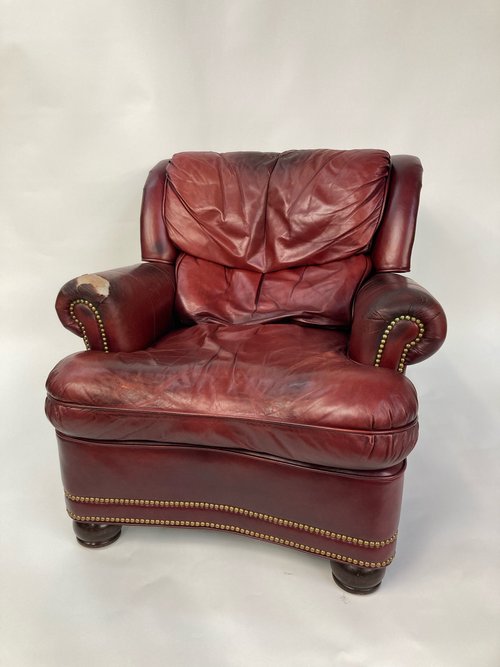The image features a vintage red leather armchair with a classic design, prominently displayed against a white background which emphasizes its aged elegance. The armchair showcases curved, robust arms and deep upholstery, indicative of both comfort and extensive use. The reddish-brown leather is worn and wrinkled, with notable creases and a small tear on one of the arms, further enhancing its character and hinting at its age. Decorative gold studs, arranged in a line along the edges and at the front of the armrests, add a touch of sophistication to the piece. The legs are short, dark, and sturdy, providing a stark contrast to the lighter hue of the leather. The armchair is slightly angled to the left, offering a full view of its textured surface and intricate details.